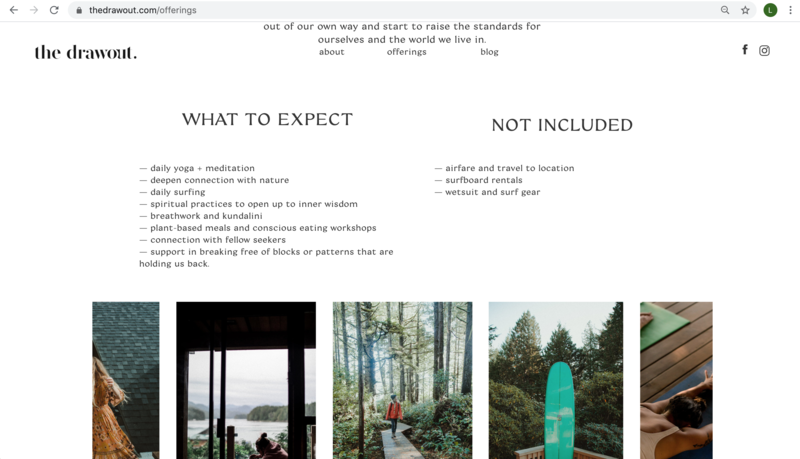The webpage screenshot is from "thedrawout.com" and features the website's taskbar prominently displaying the word "offerings." The center of the page showcases a motivational quote: "Out of our own way and start to raise the standards for ourselves in the world we live in," which is centrally aligned and easy to read. To the left, the site's name, "thedrawout," is displayed in bold, black lowercase letters.

The main section features three clear images, each depicting a serene nature scene. The first image includes a surfboard standing in front of a backdrop of towering pine trees, exuding an adventurous, outdoor spirit. The second image captures a person clad in an orange coat walking up a wooden path that meanders through lush greenery, suggesting a journey or exploration theme. The third image offers a breathtaking view of a tranquil lake surrounded by undisturbed natural landscapes, invoking a sense of peace and escape. Flanking these main images are partial glimpses of additional photos, hinting at more scenic content.

Below the images, the site details its offerings in two columns. The left column, titled "What to Expect," lists approximately eight different items or experiences provided by "thedrawout" retreats. On the right, a column labeled "Not Included" specifies three items that participants must bring themselves, such as airfare, a surfboard, and a wetsuit.